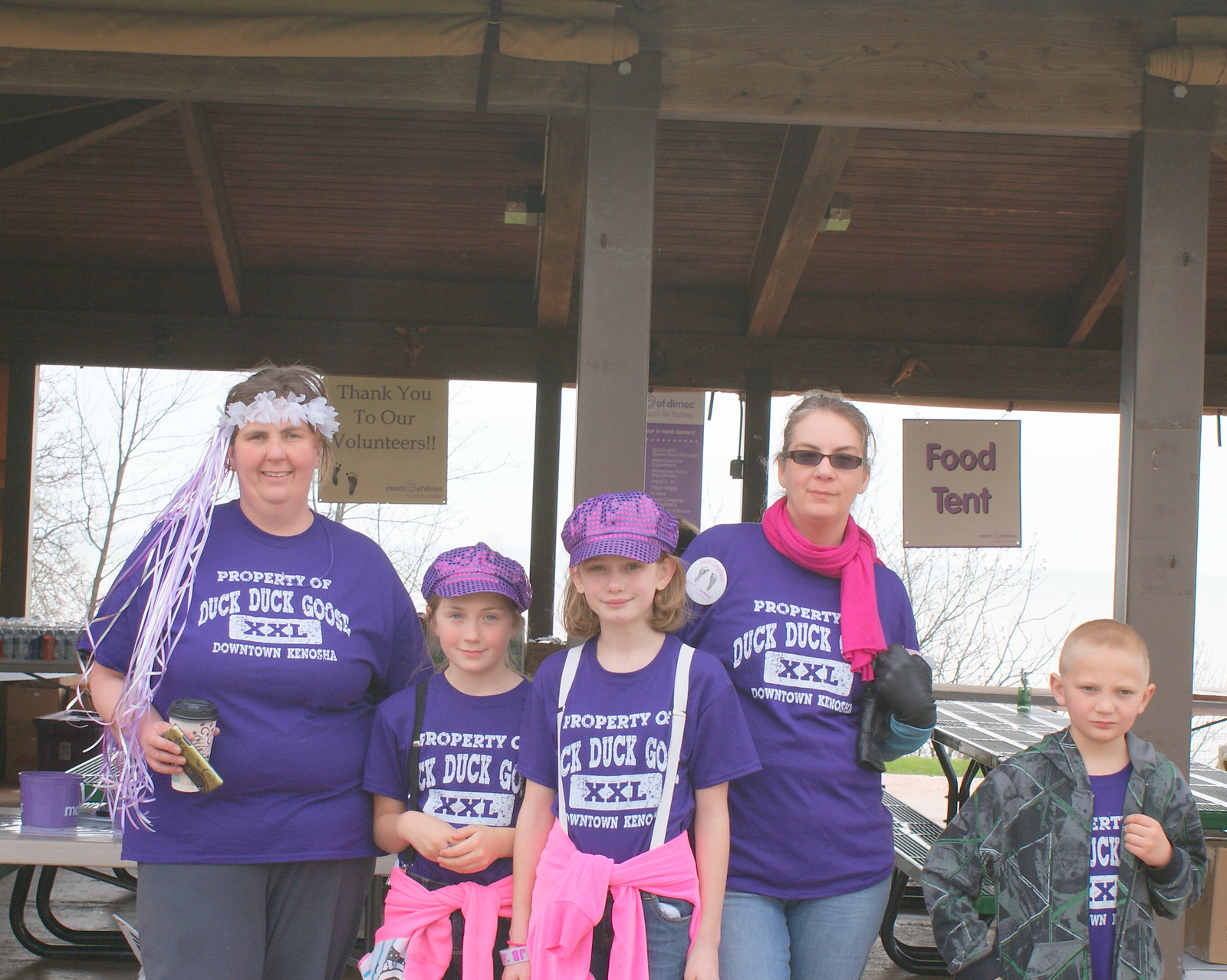In the photograph, five people stand in front of a wooden tent adorned with signs reading "Food Tent" and "Thank You to Our Volunteers," hinting at an ongoing community event. All five individuals wear matching purple shirts emblazoned with the faded text "Property of Duck Duck Goose XXL Downtown Kenosha."

On the far left is an adult woman with short or pulled-back hair adorned with a white floral wreath, the streamers cascading down her hair. She holds a paper coffee cup and something else in her right hand, and she pairs her shirt with gray sweatpants. Standing to her right are two young girls, each wearing the same purple shirt, purple hats with designs and stripes, and pink sweaters tied around their waists.

Continuing to the right, there is another adult woman, distinguished by her purple scarf and jeans. To the far right stands a young boy with a crew cut, clad in a camouflage jacket over the matching event shirt. Behind them, picnic tables are visible, reinforcing the sense of a community gathering.